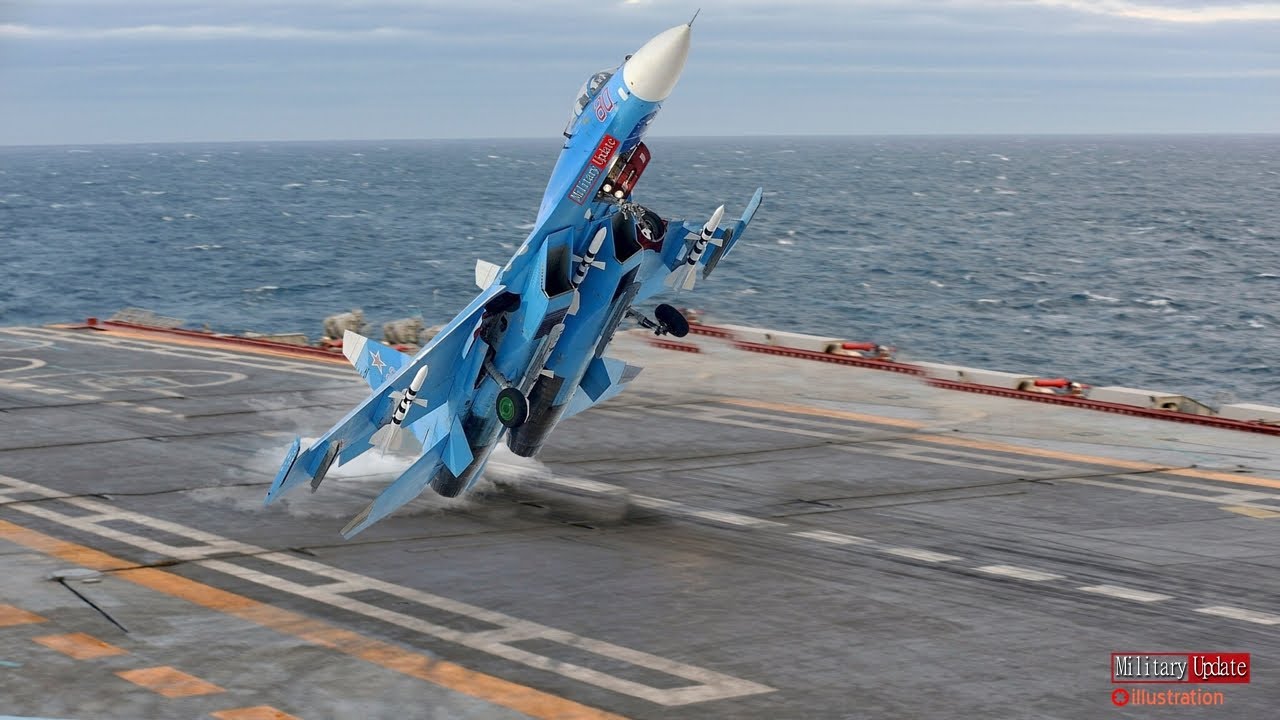The image depicts a light baby blue-colored fighter jet taking off at a steep angle, almost vertically, from what appears to be an aircraft carrier in the ocean. The aircraft, adorned with a red star with a white border on its tail and white and black missiles below both wings, features a distinctively high-positioned white front tip. The jet is captured in mid-takeoff against a backdrop of somewhat choppy ocean waves, white sea foam, and a clear sky streaked with wispy horizontal clouds. The runway on the carrier looks worn, and there are no humans visible in the image, suggesting it might be an illustration or a scene from a military-themed magazine, as indicated by the "military update illustration" text at the bottom. The overall steep ascent of the jet further heightens the dramatic effect of the scene.